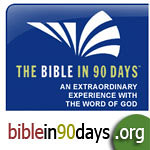This is a small, square, digital graphic, predominantly in medium blue with white text. It serves as an advertisement for a website dedicated to an immersive experience with the Word of God. At the top, bold white letters announce, "The Bible in 90 Days: An Extraordinary Experience with the Word of God," underlined by a logo composed of six brush strokes—three vertical and three angled to the right, resembling a fanned-out feather or fan. Below this, the website address, "Biblein90days.org," is prominently displayed in white text, nestled within a small green circle at the bottom of the graphic. The words "Bible" and "90" stand out in red and gold text, respectively. The overall aesthetic is cohesive, with solid blue dominating the background and one rounded edge adding a subtle design touch.